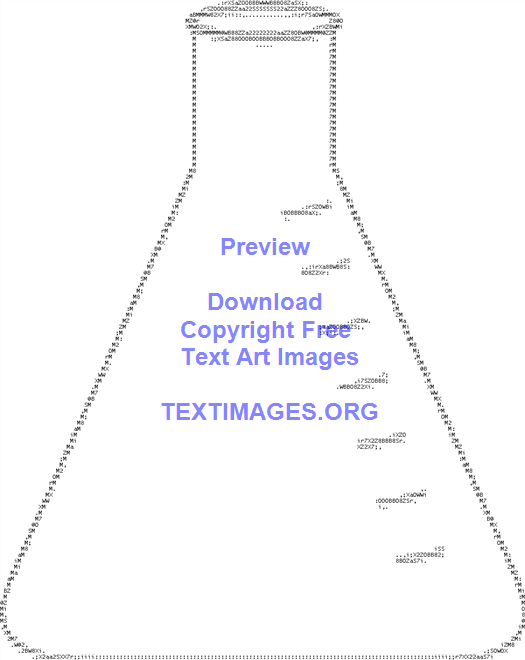The image presents a detailed text art depiction of a scientific flask, characterized by its narrow top expanding to a wider base. The flask's edges are crafted using an assortment of random characters, creating a stipple-like effect, all against a completely white background. Over the center of this intricate black and white text art, superimposed blue text reads: "Preview, Download, Copyright Free, Text Art Images." Below this, the watermark "textimages.org" is visible, indicating the source. The specific characters forming the flask are too small and blurred to discern individually.